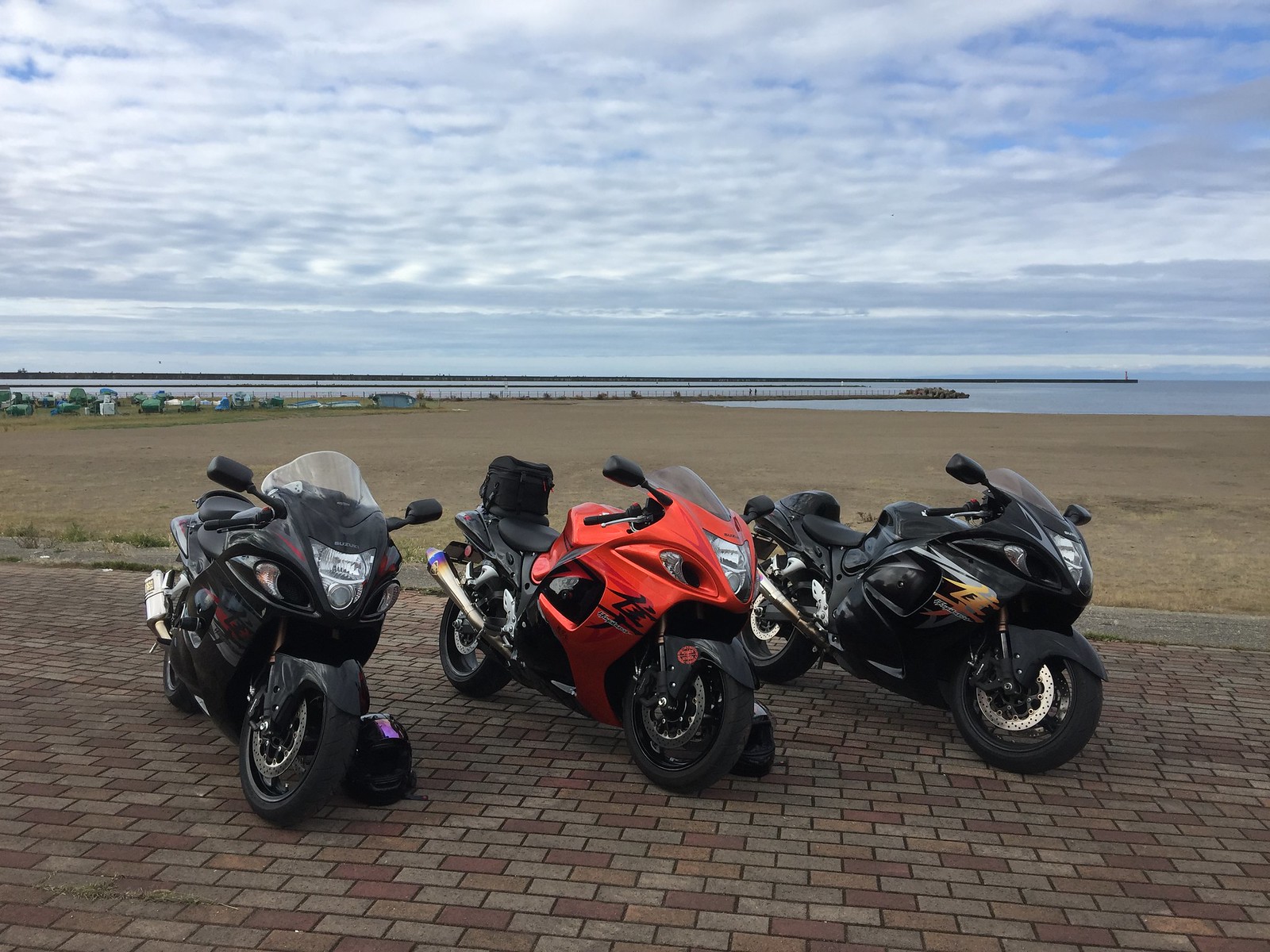On a slightly overcast day with fluffy clouds and specks of blue sky peeking through, an image captures three powerful motorcycles parked on a brick road composed of red, gray, and yellow bricks. The scene is set by a waterfront with slightly grayish water merging with a green horizon and features a long dock stretching out into the sea, a shorter dock with rocks at its end, and various small structures or tents lining the shore.

In the foreground, each motorcycle is parked with its helmet placed near its front wheel. The first bike on the left is black with crystal-clear lights and features a purple helmet beside it. The middle motorcycle is crimson orange with a black seat, a well-used silver tailpipe, black wheels, and it boasts a cooler at the back. The third motorcycle to the right is black with chrome inside wheels, black seats, and a touch of orange at the front of its motor, featuring a gold emblem. Reflective of their speed and strength, all three bikes have rearview mirrors, lights, and are positioned to face the right, adding dynamism to the scene. The setting is flat, with sand and a green area in the background, contributing to a serene yet invigorating coastal backdrop.